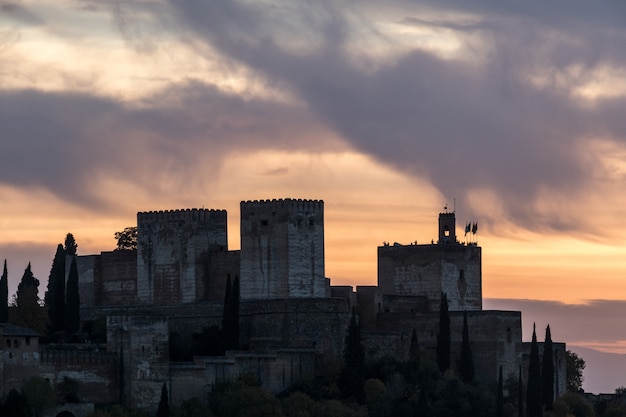At dusk, an ancient, medieval castle dominates the scene, silhouetted against an orange and gray sky. The castle, perched atop a hill, features three prominent towers, all with irregular rims at the top that historically might have served as archery battlements. The far-right tower is particularly distinguished by its flags. There are no visible lights in the castle, adding to its gloomy yet majestic aura. The sky is filled with wispy, dark gray clouds, contributing to a smoky and dramatic atmosphere. Flanking the castle are tall, slender cypress trees to the right and evergreen trees to the left, appearing as black shadows in the dim light. The entire scene, captured from a distance, highlights the imposing stone structures of the castle with their rectangular and tall silhouette, giving an impression of a fortified medieval estate amidst nature.